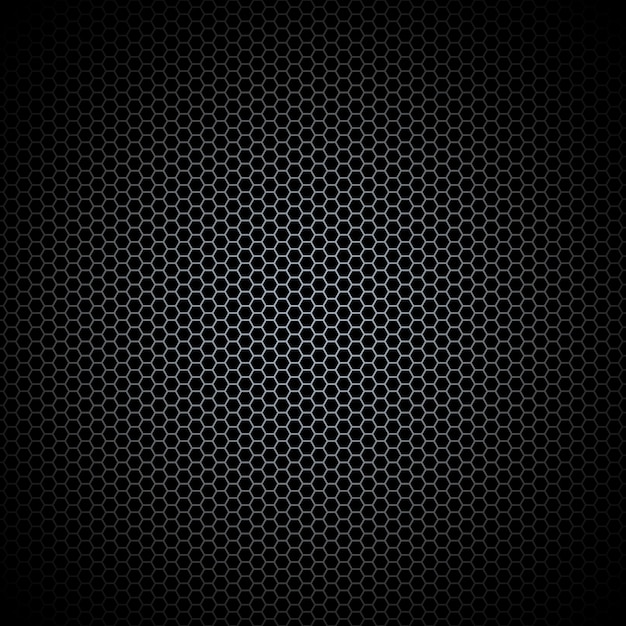The image appears to be a computer-generated graphic of a honeycomb pattern set against a deep black background. The pattern consists of octagonal cells rendered in varying shades of gray. The cells are lightest in the center, creating a focal point, and gradually darken as they extend towards the edges, where the background is completely black. This gradient effect gives the illusion of depth and makes the center appear almost three-dimensional or as if it is emerging towards the viewer. The darker edges accentuate this effect, making the honeycomb pattern seem as though it has a circular shape in contrast to the black corners. The style is modern and minimalist, potentially created using digital software like Photoshop or an AI generator, emphasizing a sleek and abstract aesthetic.